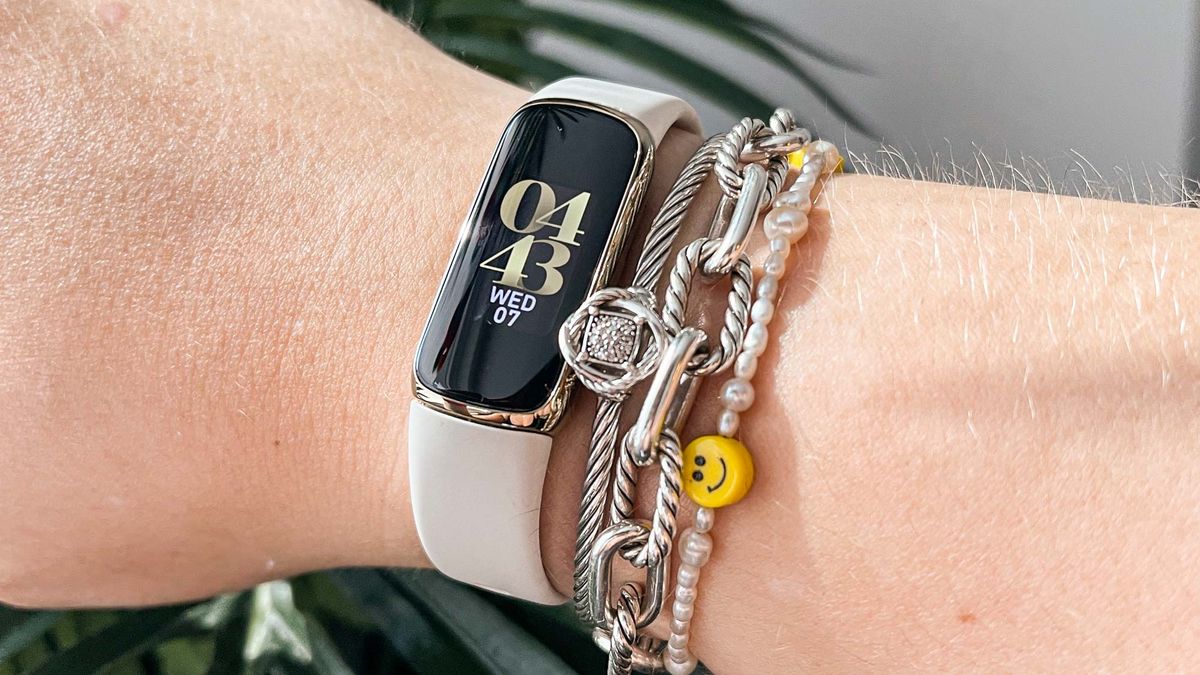This detailed, close-up color photograph captures the wrist of a fair-skinned individual, with their hand positioned on the left. The wrist wears a Fitbit-like wearable device featuring a black rectangular watch face and a cream-colored band. The display shows the time 04:43 in gold font, with the date "Wed 07" written below in white. Adorned alongside the device are multiple silver and pearl bracelets. There is a silver rope-textured bracelet with a jewel, a mixed-texture chain-link bracelet alternating between smooth and rope patterns, and a delicate pearl bracelet embellished with small smiley face trinkets. The person's arm hair is blonde, adding a subtle detail to the composition.